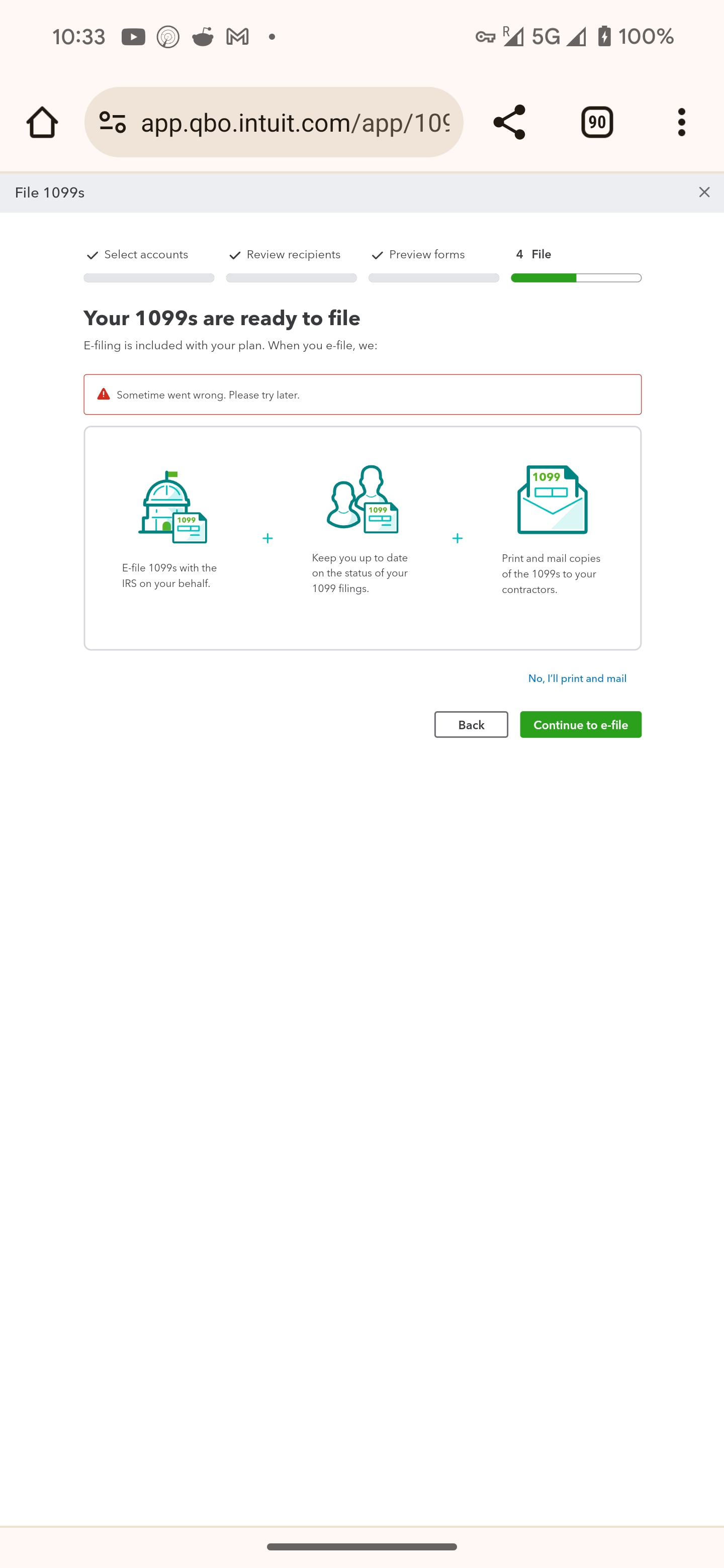Screenshot of the App Interface for Filing 1099 Forms

The screenshot captures the interface of the QuickBooks Online website (app.qbo.intuit.com/app/1099) on a mobile device. At the top of the screen, the phone's status bar is visible, showing the time as 10:33 AM, along with several notification icons: YouTube, clock, Reddit, Gmail, and a dot. Additionally, there is a key icon symbolizing a VPN connection, followed by the internet signal strength, 5G connectivity symbol, and a fully charged battery at 100%.

Below the status bar lies the internet browser interface. On the left side is the home button, followed by the URL address bar displaying the website address. Positioned next to the address bar are options to share the page and a box displaying the number of open tabs, which shows "99" in this instance. Furthermore, there is a three-dot menu icon for additional browser settings.

The main content of the screenshot shows a gray bar at the top labeled "File 1099," with an 'X' icon in the top right corner for closing the notification. The main section of the page is presented on a simplistic, clean white background. It informs the user that their 1099s are ready to file. At the bottom of the screen, there is a bright green button labeled "Continue with Filing" and an option for going back via a back button.

This detailed view provides a comprehensive understanding of the interface and the various elements visible on the screen for the task of filing 1099 forms.